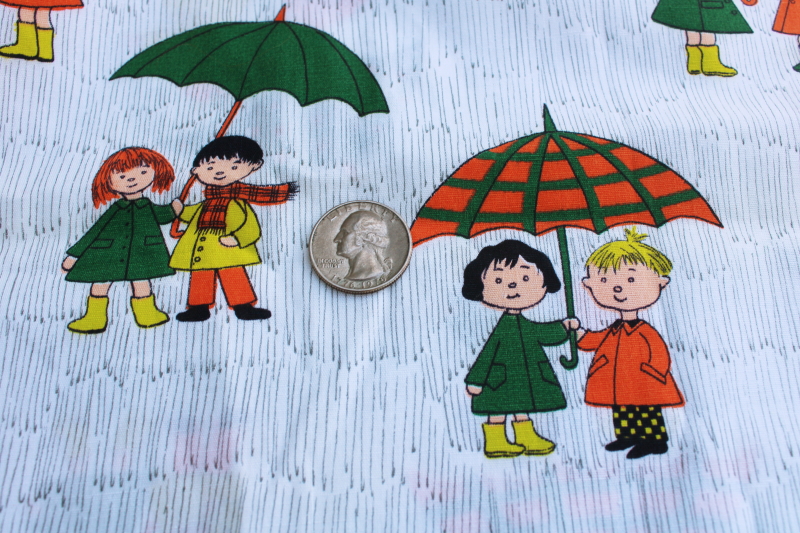This image depicts a horizontally aligned rectangular piece of artwork resembling a child’s blanket with a white background adorned with thin dark gray zigzag patterns. At the center lies a silver quarter, heads up, emphasizing the scale. 

On the left side of the artwork, there are two cartoon-like characters: a girl with short red hair, a green coat, and yellow boots, holding a green umbrella; she stands next to a boy with short black hair, dressed in a yellow jacket, a plaid red scarf, and orange pants. 

To the right of the quarter, there is another pair of children. The girl, sporting short black hair, wears a similar green coat with yellow boots, while the boy beside her has blond hair and is dressed in an orange jacket and black pants with yellow polka dots. They hold an umbrella that is orange with green stripes. The upper corners of the image feature additional patterns and more yellow rain boots can be seen, enhancing the whimsical rain-ready theme.